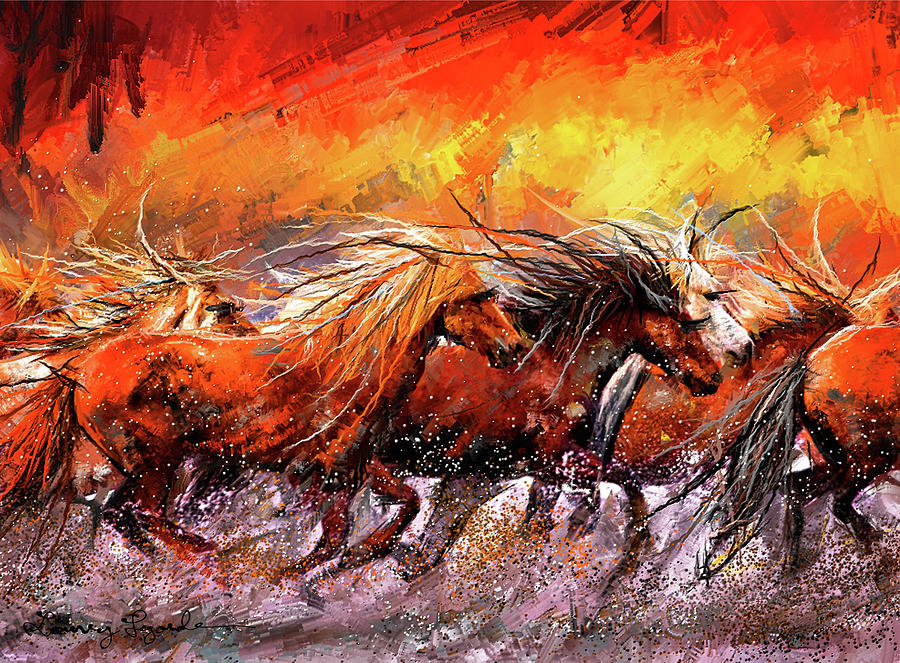This captivating painting depicts a group of wild horses galloping through what appears to be a body of water. The background is a dramatic blend of red, orange, and yellow hues, evoking the imagery of a blazing fire. The fiery tones cast a mesmerizing reflection on the water's surface, enhancing the scene's intensity. In the foreground, splashes of water add a dynamic sense of movement as the horses charge forward. Each horse is beautifully detailed: their manes, long and flowing, vary in shades from blonde to brown, with one striking white horse among them. The unkempt appearance of their manes suggests their wild nature, giving the impression that these majestic creatures are fleeing from an encroaching fire into the safety of the water.